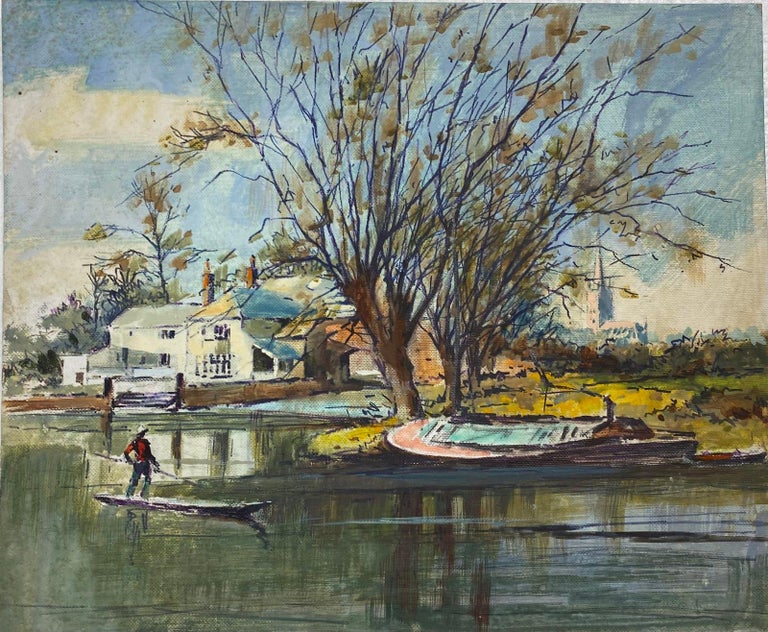This watercolor painting captures a serene nature scene with a variety of elements contributing to a rich and detailed landscape. In the background, a house with a blue roof and two chimneys is partially obscured by distant trees. There is a large, grassy field to the right of the house, which appears golden, indicating it might be spring when leaves are beginning to regrow. Central to the composition are two large trees with sparse foliage, extending their branches towards a sky tinged with gray, blue, and white hues, indicating a mix of clouds. Beneath these trees, a river cuts through the landscape, reflecting the trees and the sky. On the right side, a small boat is moored along the riverbank. To the left, a man in a red shirt and blue jeans stands in another boat, using a long paddle to navigate the water. Behind the house, a church steeple, reminiscent of classic chapel architecture, punctuates the skyline, adding a historic character to the scene. The reflective water, accented by the watercolor's light and dark shades, ties together the natural and man-made elements, creating a peaceful tableau.